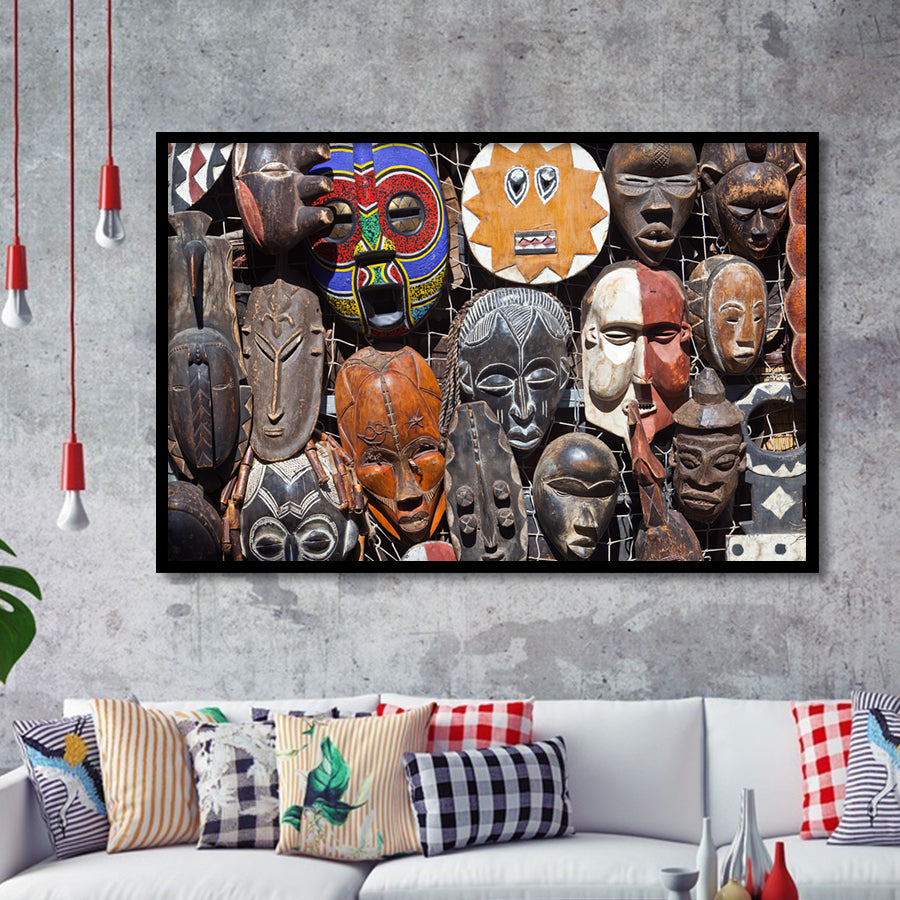This photograph captures a cozy living room setting, centered around a large, vibrant piece of artwork mounted above a pristine white couch replete with an assortment of colorful cushions. The artwork, a striking collage of various tribal masks, predominantly seems to depict African masks, though some suggest influences from Mayan or Aztec cultures. The masks are diverse in shapes, sizes, and colors; most are fashioned from dark, unfinished wood, while one particularly eye-catching mask features an array of bright colors including blue, red, yellow, and green.

The white couch below the artwork is adorned with a variety of cushions, creating a lively contrast against the monochromatic wall. These cushions include a black and white striped pattern, a couple of red and white checkered ones, a flannel-like black and white cushion, and a pair of purple cushions.

To the left of the artwork, a distinctive light fixture hangs, featuring three bulbs suspended from a striking purple wire, each encased in a red cover, casting a warm glow over the scene. Additional decor includes a collection of colorful vases in hues of silver, red, white, gray, and yellow, arranged on a table near the couch, adding to the eclectic yet harmonious aesthetic of the room.